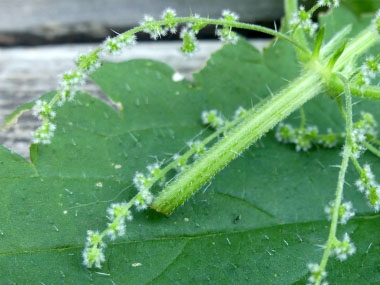This detailed nature photograph captures a vibrant scene of a bright green plant resting on a darker, frayed-edged leaf. The image is highly magnified, revealing the plant’s fuzz-covered stem with three smaller stems branching off, each adorned with tiny clusters of white, fluffy flowers. The contrast between the lively, light green hue of the plant and the muted, heavier tone of the underlying leaf provides a striking visual, highlighting the intricate textures and delicate structures of both the plant and the leaf. The leaf itself shows an irregular, torn edge and visible veins, adding to the natural complexity and detail of the image.